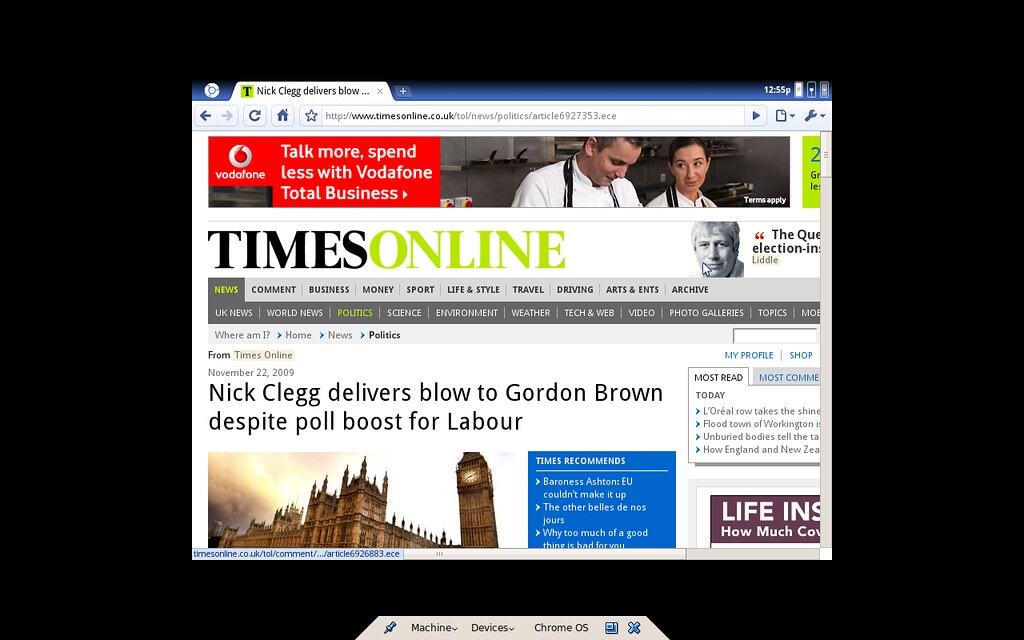In this detailed image, we observe a webpage from the Times Online news outlet. The URL visible in the browser tab reads "https://www.timesonline.co.uk" followed by a specific article link "https://news.politics.article6927353.ese". The webpage is adorned with various sections and categories such as "Talk more, spend less with Vodafone" and "Total Business," showcasing advertising and promotional content. The navigational menu includes labeled sections for "Times Online," "News," "UK News," "World News," "Politics," "Science," "Enrollments," "Weather," "Tech and Web," "Video," "Photo Galleries," "Topics," and "Where Am I."

The main article displayed on the page is from the Politics section, dated November 22, 2009. The headline reads, "Nick Clegg delivers blow to Gordon Brown, despite poor boost for Labour," indicating a significant political event covered by Times Online. This detailed and comprehensive layout provides a clear snapshot of the diverse content and navigational structure featured on the Times Online news outlet's webpage.